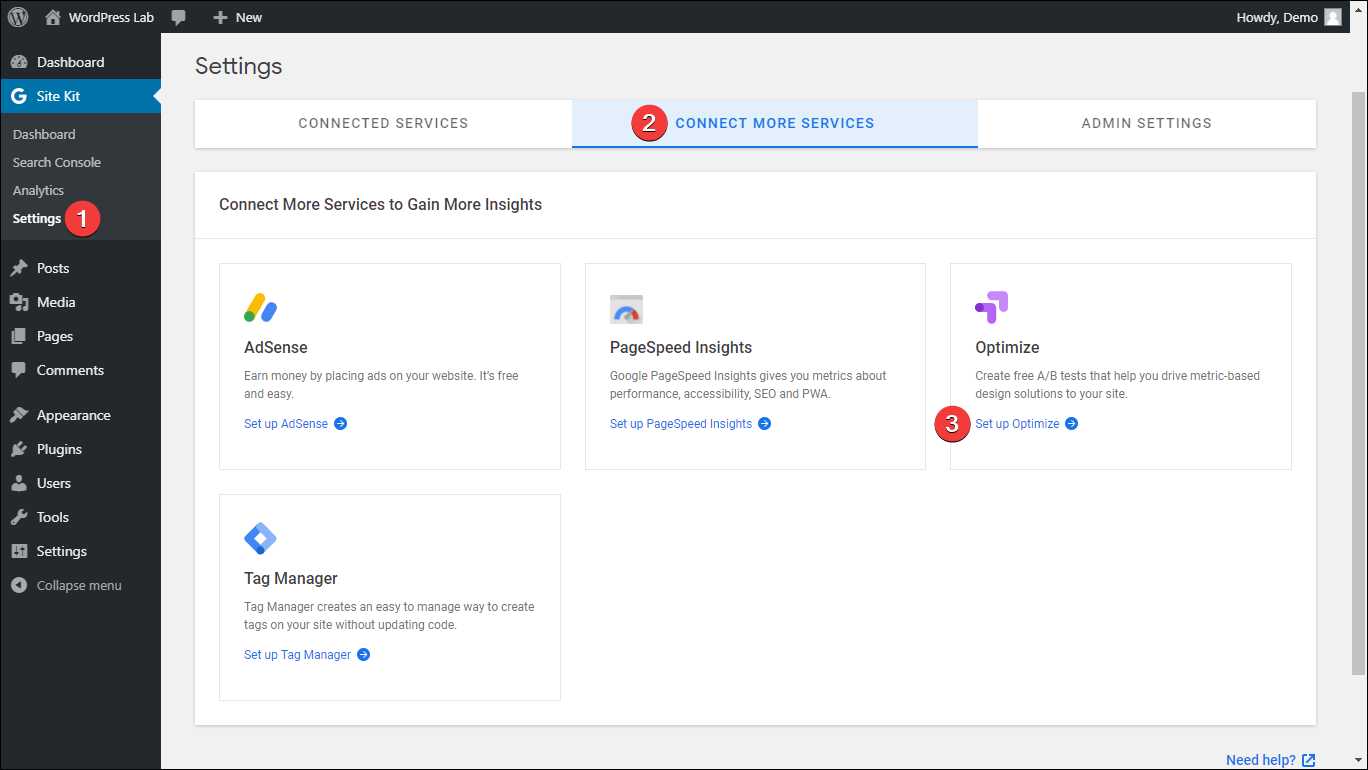Screenshot of a WordPress Dashboard

This screenshot captures a WordPress dashboard interface. A blank bar stretches across the top, featuring essential navigation elements. On the far left, the WordPress logo (WB) is prominently displayed, followed by a home button labeled "WordPress Lab." 

Towards the right of the top bar, there is a series of functional buttons: a chat button, a "Plus New" button for creating new content, and finally, a user greeting "Howdy, Demo" accompanied by a default user icon on the far right.

On the left side of the screenshot, a dark grey/black vertical sidebar houses key administrative options. From top to bottom, the sidebar menu includes:

- Dashboard
- Site Kit
  - Dashboard
  - Search Console
  - Analytics
  - Settings

Following this section, the menu continues with options for:

- Posts
- Media
- Pages
- Comments
- Appearance
- Plugins
- Users
- Tools
- Settings
- Collapse Menu

Each menu item is presented as a single word per button, per line, stacked vertically to facilitate easy navigation.